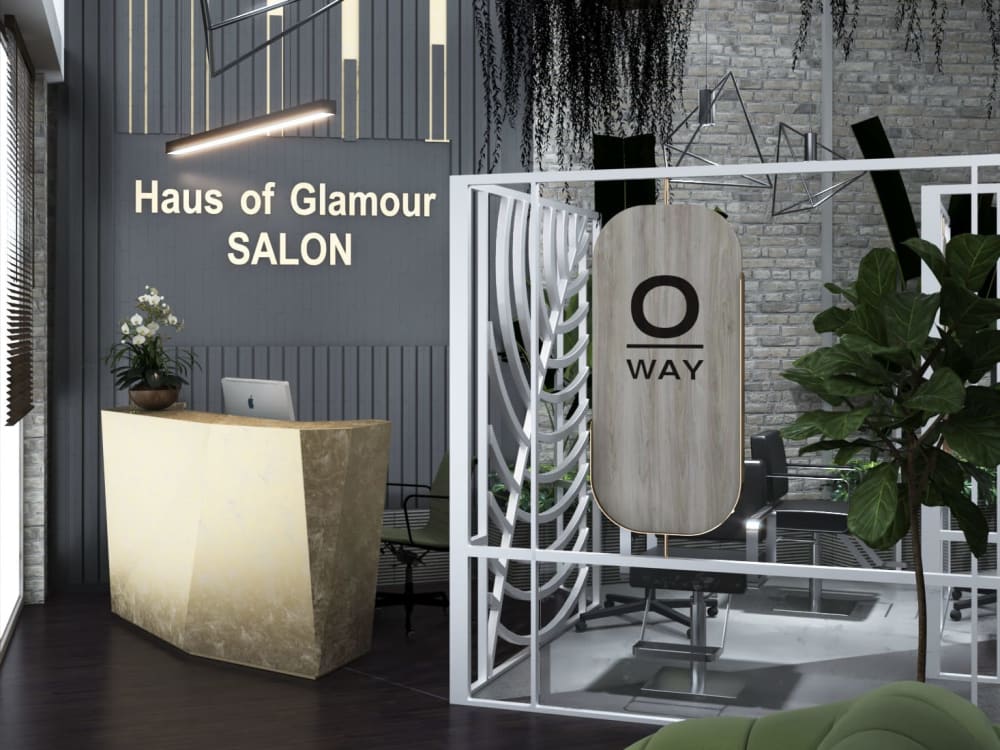This image showcases the interior of the House of Glamour Salon, emphasizing its modern and elegant design. The walls feature a smooth dark grey on one side and a light grey brick on the other, contrasting beautifully with wood and metal accents. The floor is dark and reflective, enhancing the salon's contemporary aesthetic. Dominating the entrance is a light marble reception desk, adorned with a chair, an Apple computer, and a sophisticated flower arrangement. A bright sign above the desk boldly displays "House of Glamour Salon." Adjacent to the reception area, a lush green plant in a white pot adds a touch of nature. A white structure nearby contains an oval sign inscribed with "OAE" or "OA." Transitioning into the salon area, you find two hairstyling stations, separated by dividers that create an open yet defined space. Hanging mirrors with the inscription "Zero Way" or "O-Way," along with strands of suspended ferns that descend from the high ceiling, contribute to the salon’s airy and spacious feeling.